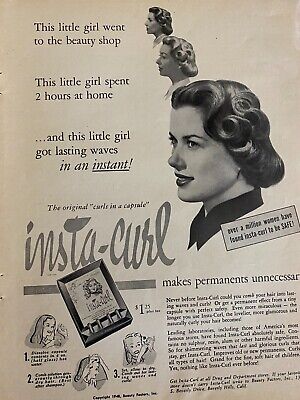The advertisement from the 1940s or 1950s features a black and white poster for a product called Insta-curl. Dominating the top of the poster are three vertically stacked, black and white cutout photographs of women with short, wavy hair. Each photograph is accompanied by the caption: “This little girl went to the beauty shop,” “This little girl spent two hours at home,” and “This little girl got lasting waves in an instant.” On the right side of these photographs, the name "Sophie" suggests the model's identity.

At the center left of the poster, the name "Insta-curl" is prominently displayed in large, cursive font, further emphasized by the tagline, "The original curled in a capsule," situated above it. Below this, a paragraph begins with the bolded title, "Makes permanence unnecessary," though the remainder of the text is too small to read clearly. The ad’s white background shows signs of aging, with yellowing adding a touch of vintage charm.